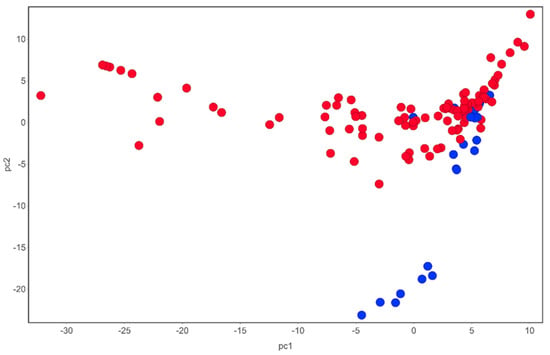The image depicts a detailed scatter plot graph, with the x-axis labeled as PC1 and ranging from -30 to 10, and the y-axis labeled as PC2, spanning from -20 to 10. The graph features red and blue dots indicating different data points. Blue dots begin at approximately (-5, -20) on the graph and cluster around that region, extending sporadically up to (5, 5). In contrast, the red dots are more widespread, beginning around (-34, 4) and stretching across the entire graph, reaching up to (14, 10). There are notably more red dots than blue dots, with the red dominating predominantly in the upper regions and distributed broadly across the chart, indicating a broader range of variability or measurements for the red data points compared to the blue.